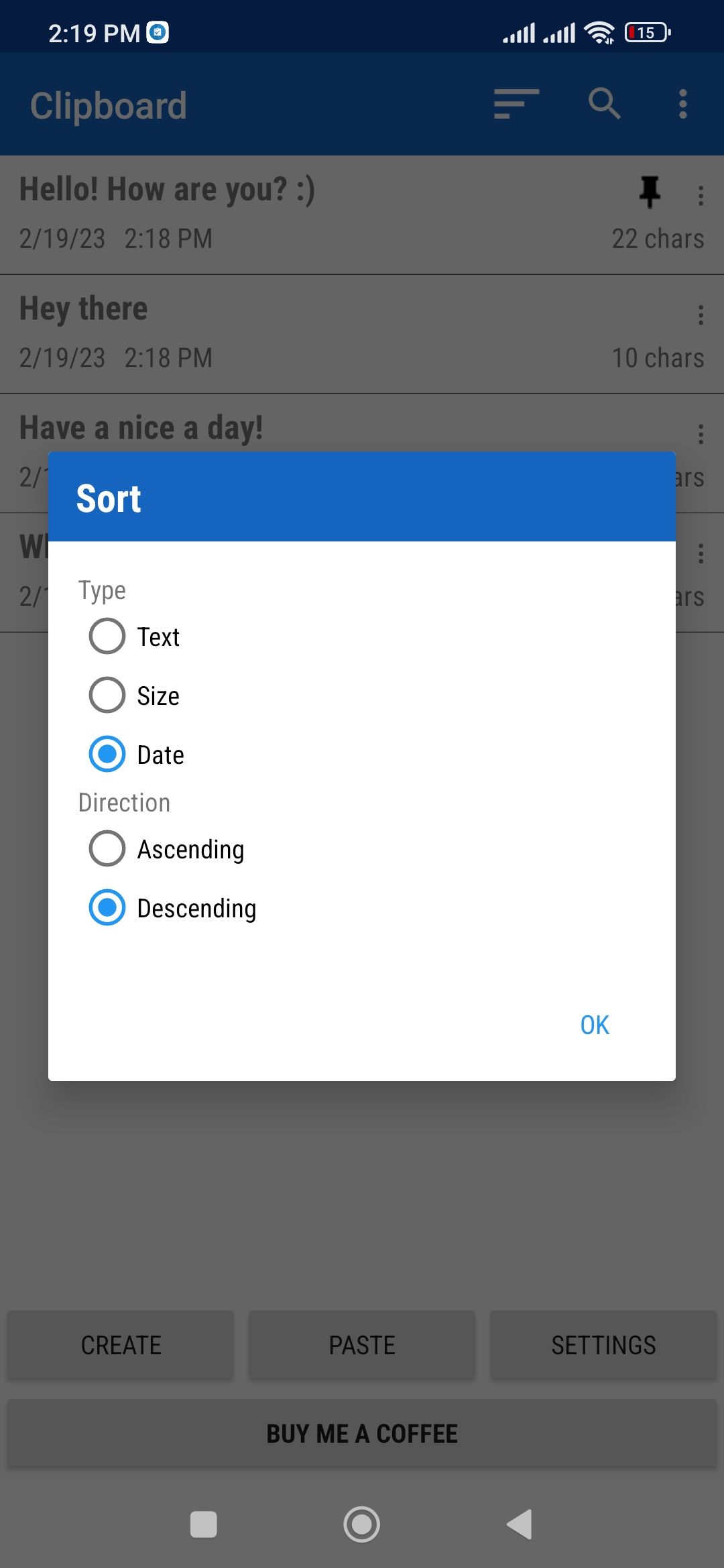This is a detailed capture of a smartphone screenshot featuring various user interface elements. The top border is dark blue, displaying a time stamp of 2:19 p.m. on the left side, a strong Wi-Fi signal, and a battery level at 15% on the right side. Directly below this, there's a lighter blue border holding a clipboard icon and three vertical lines of differing lengths.

The main part of the screen is predominantly white, starting with a section that reads "Hello! How are you?" accompanied by a smiley face emoji, a pin icon to the right, and three gray dots. Underneath, there's a timestamp dated 2-19-2023 at 2:18 p.m., followed by the number "22 shars" on the right. Below this is another message, "Hey there!” with a timestamp of 2-19-2023 at 2:18 p.m., along with "10 shars" and three dots to the right. Further down, there's a message stating, "Have a nice day!" with an exclamation point, though the date and "shars" count are not visible.

At the lower section of the screen, a pop-up box with a blue border appears. Within this box, the word "Sort" is prominently displayed in white text. Below "Sort," white bubbles indicate different sorting options: "Text," "Size," "Date" (which is selected), and under "Direction," "Ascending" (unchecked) and "Descending" (checked). An "OK" button sits at the bottom right of this pop-up.

The main screen, partially obscured by a gray shade, displays three functional buttons at the bottom: "Create," "Paste," and "Settings." Below these, there's a box with black text reading "Buy me coffee." Finally, near the bottom, standard navigation buttons include a "Stop" button, a "Home" button, and a left-facing arrow button, completing the interface layout.